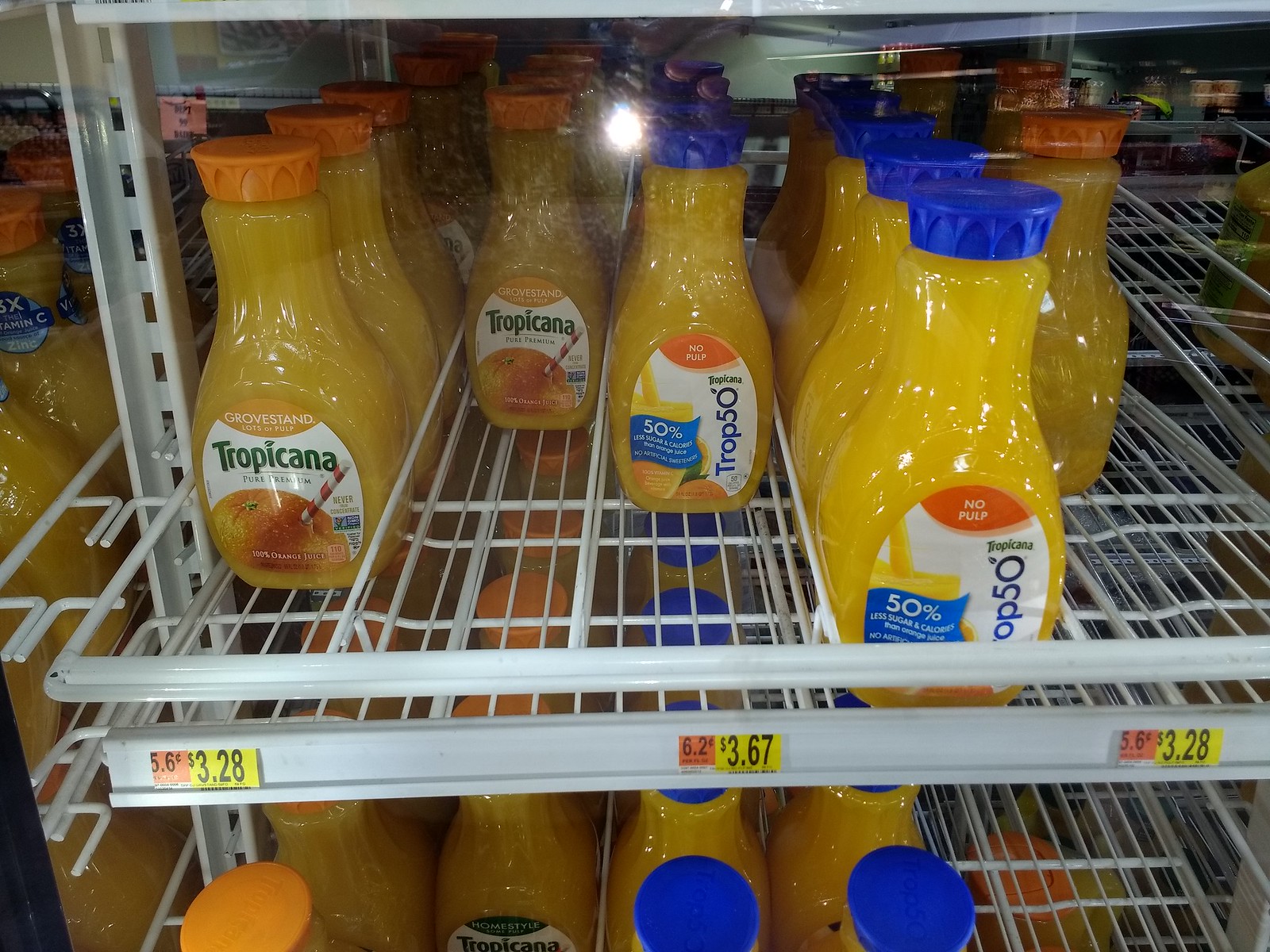A meticulously organized display of orange juice bottles sits on a wire rack shelf within a grocery store cooler. The shelf features individual lanes tailored to each type of bottle. From left to right, the arrangement starts with Tropicana, followed by Grove Stand, then another Tropicana, and another Grove Stand further back. The vibrant orange juice fills the clear, see-through bottles, accentuated with bright orange lids. The front labels showcase an image of an orange adorned with a whimsical red and white barber pole-style stripe inserted into it. 'Tropicana' is prominently written in green. To the right of the Tropicana bottles stands Prop 50, also containing orange juice in a transparent bottle, but with a distinguishing blue lid. Its label clearly states 'No Pulp' in bold white text set against a striking red background. Price tags are displayed just below these bottles, while an additional row of assorted juice bottles resides on the shelf beneath.